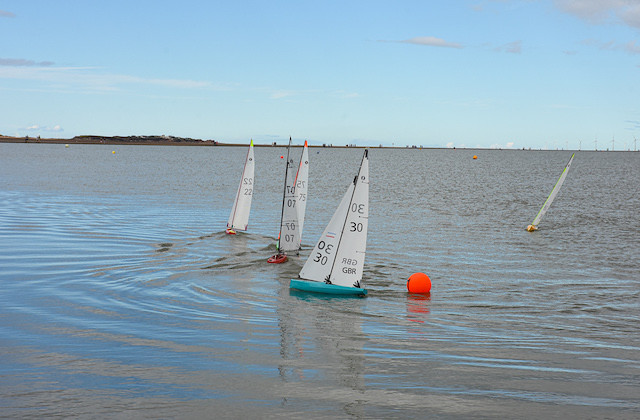In this vibrant and sunny photograph, four miniature sailboats — seemingly from a radio sailing club — skim across a large body of water near the shore. The boats are easily identifiable by their distinct bottom colors: the closest has a teal bottom, another to its left a reddish bottom, and further left, two boats with cream-colored bottoms. Stretching into the horizon, the water presents a serene yet expansive view edged by a distant island and possibly some windmills. The boats' white sails are adorned with numbers, notably "30-30", "70-70", and "75-75", with the initials "GBR" visible, suggesting affiliation with Great Britain. A few orange buoys and a red bobber float nearby, adding to the scene's nautical charm. The sky above is a radiant blue, dotted with a scatter of fluffy clouds, reinforcing the day's clarity and calmness. There’s also a subtle glimpse of the sandy shore with gentle waves, grounding this picturesque maritime snapshot.